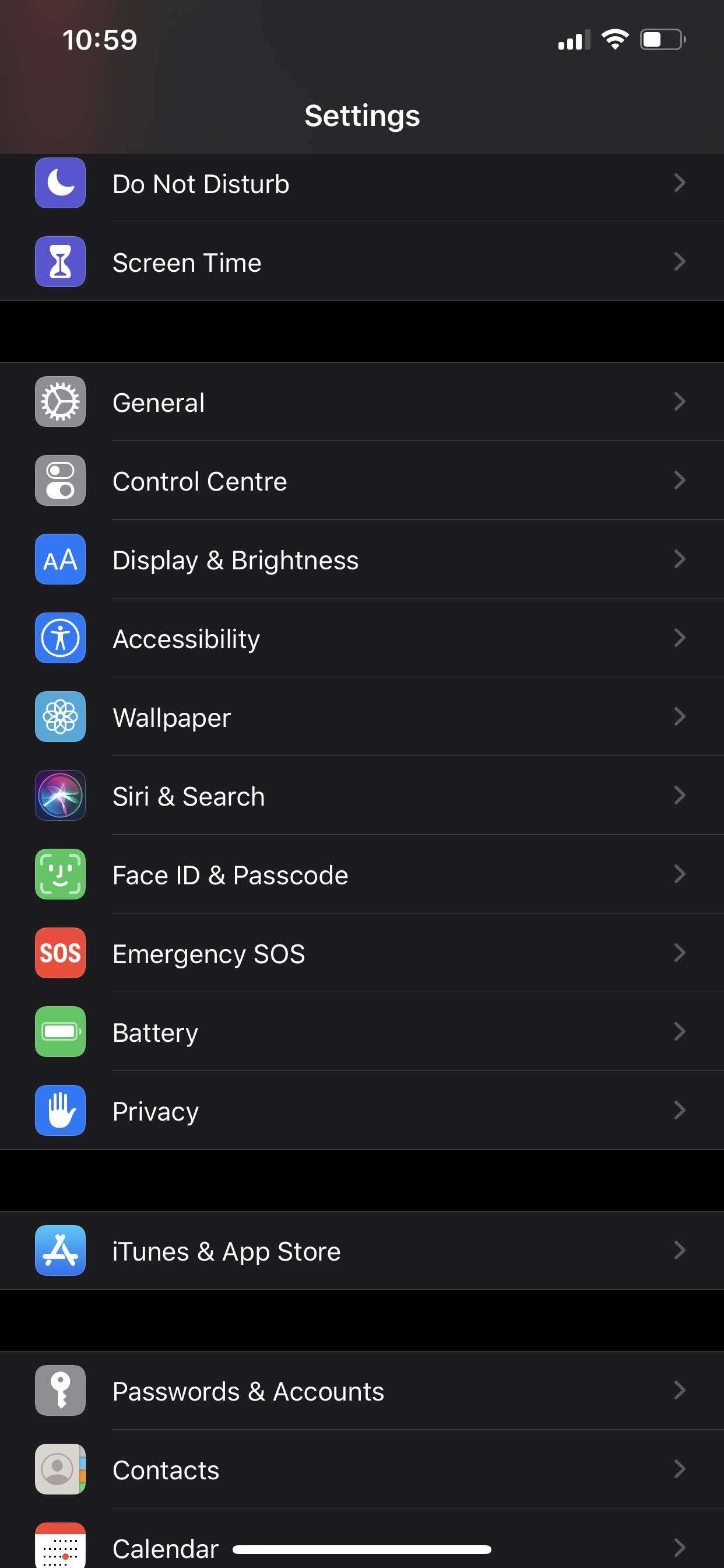This image depicts a smartphone's settings page, prominently featuring a black background with white text. At the top of the screen, the time is displayed in white, reading "10:59." Additionally, status indicators for cellular signal, WiFi connectivity, and battery life, along with signal bars, are visible.

The page is subdivided into several sections, each represented by distinct icons and backgrounds:

- **Do Not Disturb**: No icon specified.
- **Screen Time**: No icon specified.
- **General**: Identified by a gear icon.
- **Control Center**: Distinguished by a gray background with two buttons.
- **Display & Brightness**: Marked with two large A's.
- **Accessibility**: Featuring a blue background with an icon of a person with arms outstretched.
- **Wallpaper**: Noted with a light blue background.
- **Siri & Search**: Showing a colorful circular icon.
- **Face ID & Passcode**: Characterized by a green icon.
- **Emergency SOS**: Highlighted with a red background and an SOS icon.
- **Battery**: Represented by a green background and a battery icon.
- **Privacy**: Denoted by a blue background and a white hand icon.
- **iTunes & App Store**: Evident by the blue App Store icon resembling the letter "A."
- **Passwords & Accounts**: Represented by a passkey icon.
- **Contacts**: No icon specified.
- **Calendar**: Indicated by the outline of a red and white calendar.

This detailed organization and vivid iconography provide a comprehensive overview of the phone's settings menu, making it easy for users to navigate and customize their device.